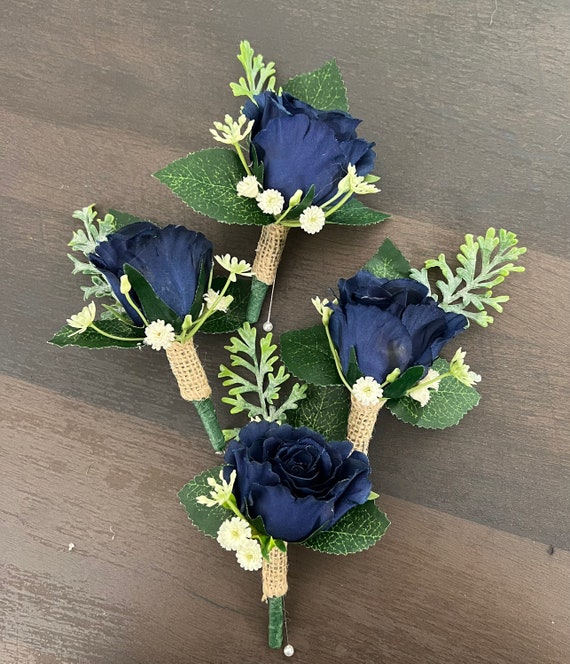This photograph showcases a meticulously crafted arrangement of four corsages, positioned in a diamond shape at the center of a dark brown, wooden table with visible slats. The corsages are composed of dark blue, artificial roses, each accompanied by three dark green leaves and accented with tiny white flowers reminiscent of baby’s breath, as well as yellowish-green leaves. The long green stems of the corsages are carefully wrapped in a light tan burlap-like fabric. Additionally, each corsage features a white string adorned with a pearl-like bead, dangling at the bottom. Despite being crafted from identical materials, each corsage is uniquely positioned, adding to the visual interest and charm of the arrangement.